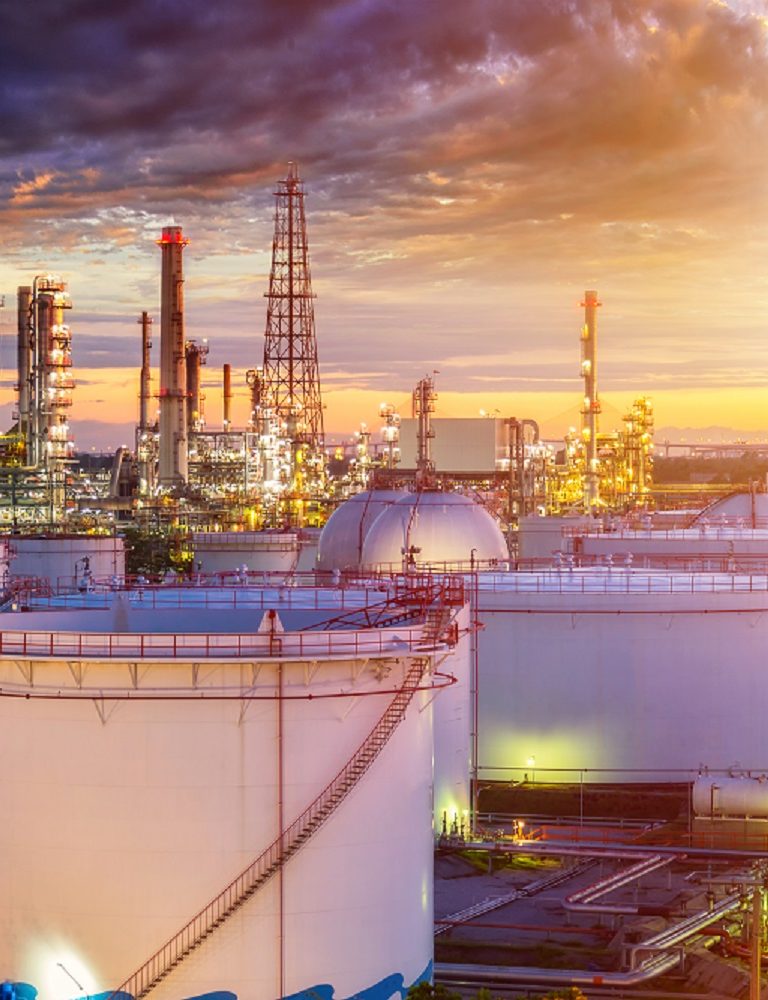In this color photograph, we see a sprawling industrial complex, possibly an oil refinery or chemical factory, captured during the early moments of sunrise or the onset of twilight. The scene is dominated by large, white cylindrical tanks, one of which on the bottom left features a staircase spiraling up its side. To the right of this tank, there's a flat, rectangular platform close to the camera. As our gaze moves upwards and into the middle of the image, a myriad of towering structures and equipment becomes visible, all illuminated by yellow lights. These include cylindrical and metal-bar towers that extend vertically. The sky in the background is a dramatic gradient, transitioning from a warm gray and orange near the horizon to darker gray and blue clouds overhead. The right side of the sky exhibits lighter hues with hints of orange, adding an atmospheric contrast to the industrial silhouettes below, enhancing the overall ethereal quality of the photograph.